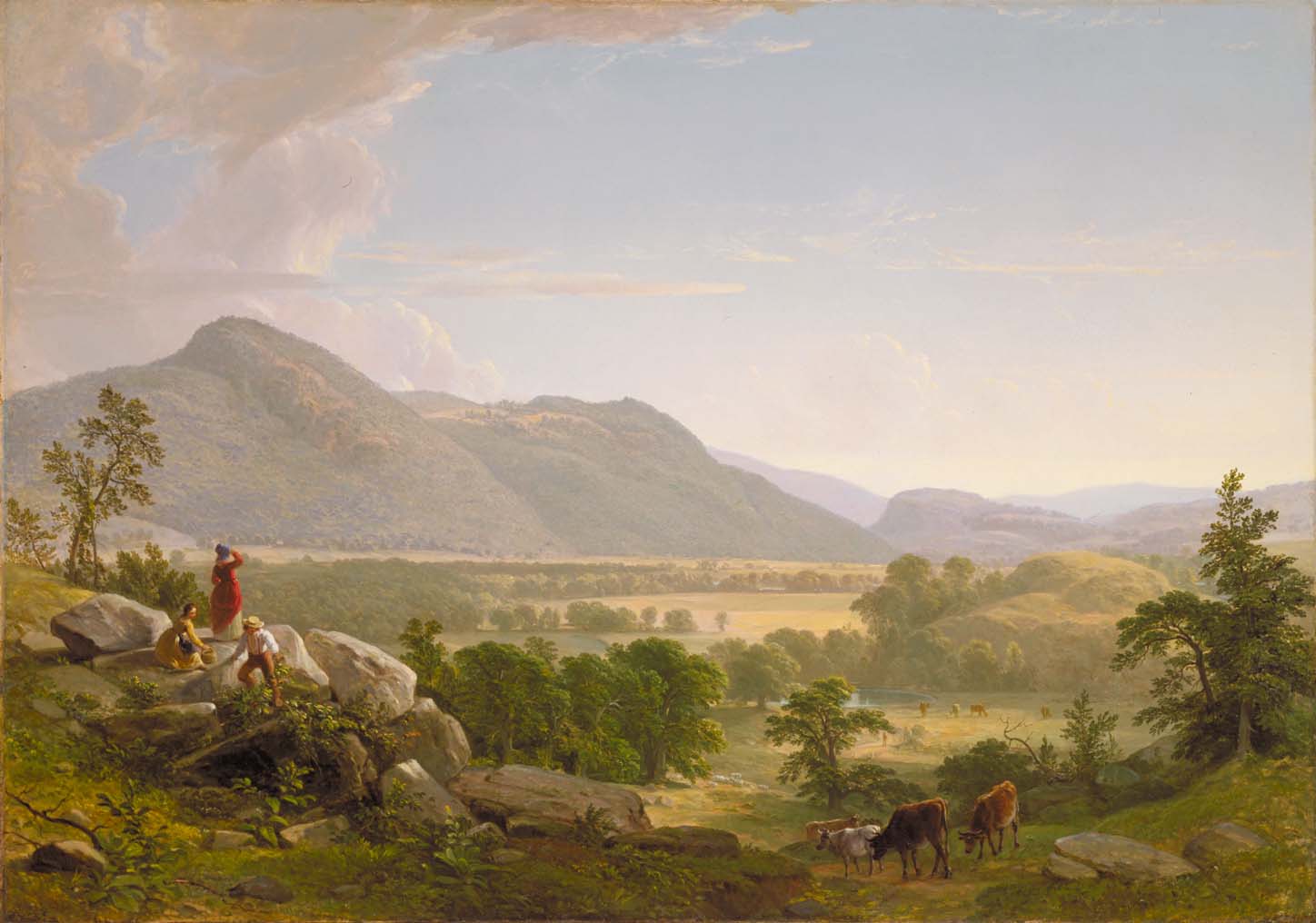The painting depicts a serene, bucolic mountain scene reminiscent of the landscapes in "The Sound of Music." The terrain is lush with greenery, featuring hills and mountains in the distance with layers of green grass and numerous trees throughout the foreground. Notably, there is a clear blue sky with patches of haze and clouds. 

In the foreground, there are four cows and horses, with a couple more spotted in the background, adding a pastoral element to the scene. The animals, mainly brown with a few white ones, are mostly positioned at the bottom right of the painting. To the bottom left, there are several rocks and bushes, where we find a woman in a vibrant red dress, her hand raised as she gazes out toward the horizon. Nearby, two other figures, appearing slightly old-fashioned and less clear, accompany her; one wears a hat.

The painting has a slightly hazy quality, indicative of an older or intentionally stylistic piece, rather than a crisp photograph. The mixed palette includes various shades of green, yellow, tan, brown, red, blue, and gray, contributing to the rich and lively atmosphere of this outdoor midday setting.